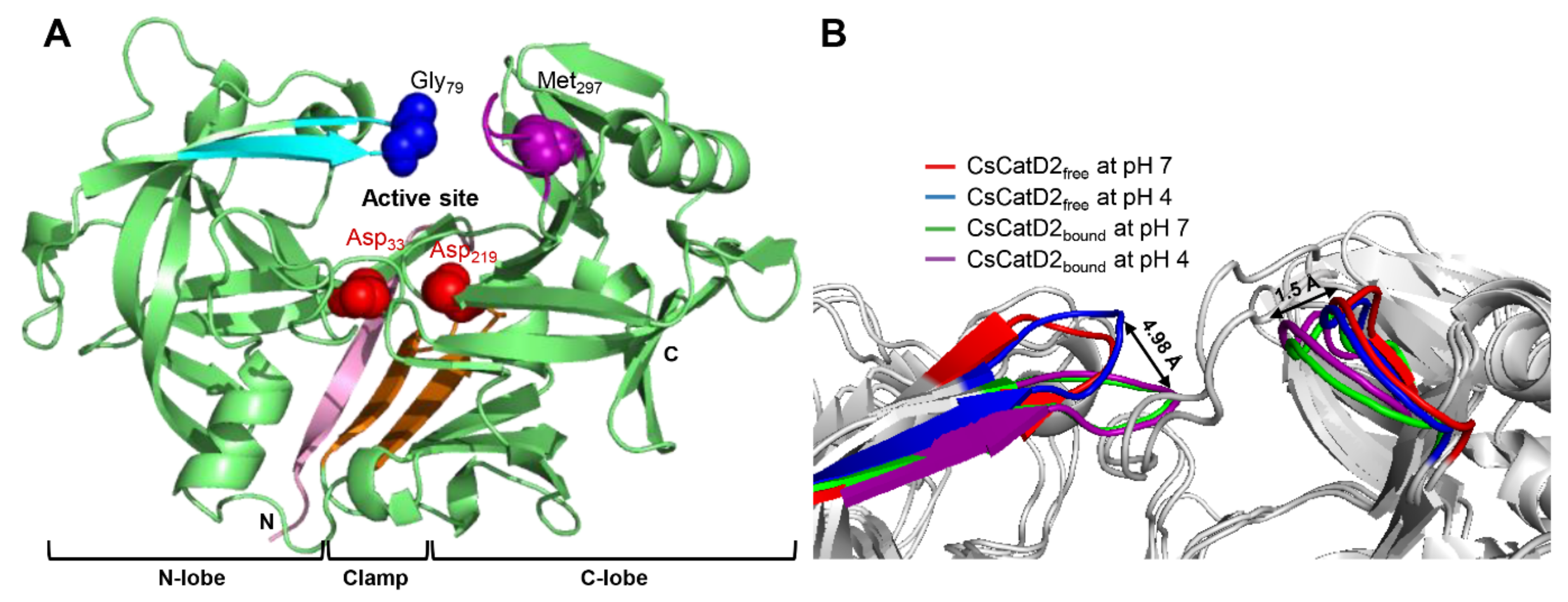The image is a scientific diagram against a white background. It is divided into two sections labeled "A" on the left and "B" on the right. Section A features green ribbon-like structures intertwined with raspberry-like red dots, blue and purple spheres, and various labels including GLY79, MET297, ASP33, and ASP219. Additional notes such as ENLOBE, CLAMP, and CELOBE are visible at the bottom. Section B shows a schematic with thin white tubes and metal wires accompanied by diverse colored wires in red, blue, green, and purple. This section includes labels such as CSCATD2 free at pH 7, CSCATD2 free at pH 4, CSCATD2 bound at pH 7, and CSCATD2 bound at pH 4. A key to the right explains the color coding.